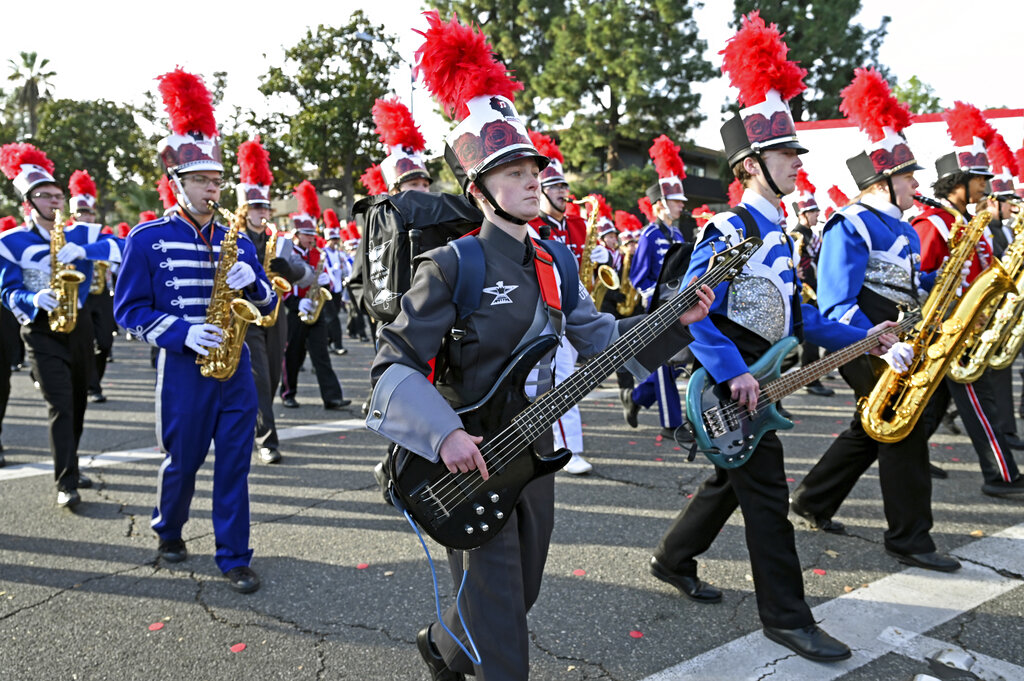This full-color image captures an outdoor scene of a marching band in a parade. The parade takes place on a blacktop roadway, featuring visible cracks and white markings for pedestrian walkways and vehicle lanes. The sky above is overcast, casting a white hue, while tall, green trees line the background, adding a touch of nature to the scene.

The marching band members, marching in unison, wear a variety of standard marching band uniforms. Some members sport royal blue tops with white detailing and black pants, while others wear gray uniforms. The front line of the band includes musicians playing bass guitars and trombones, with numerous saxophone players situated in the back rows.

Each band member wears a tall, white hat adorned with a black rim, a black neck strap, a rose print, and a bright red fluffy feather emerging from the top. The image vividly showcases the diverse attire and unity of the band as they parade along the asphalt road.